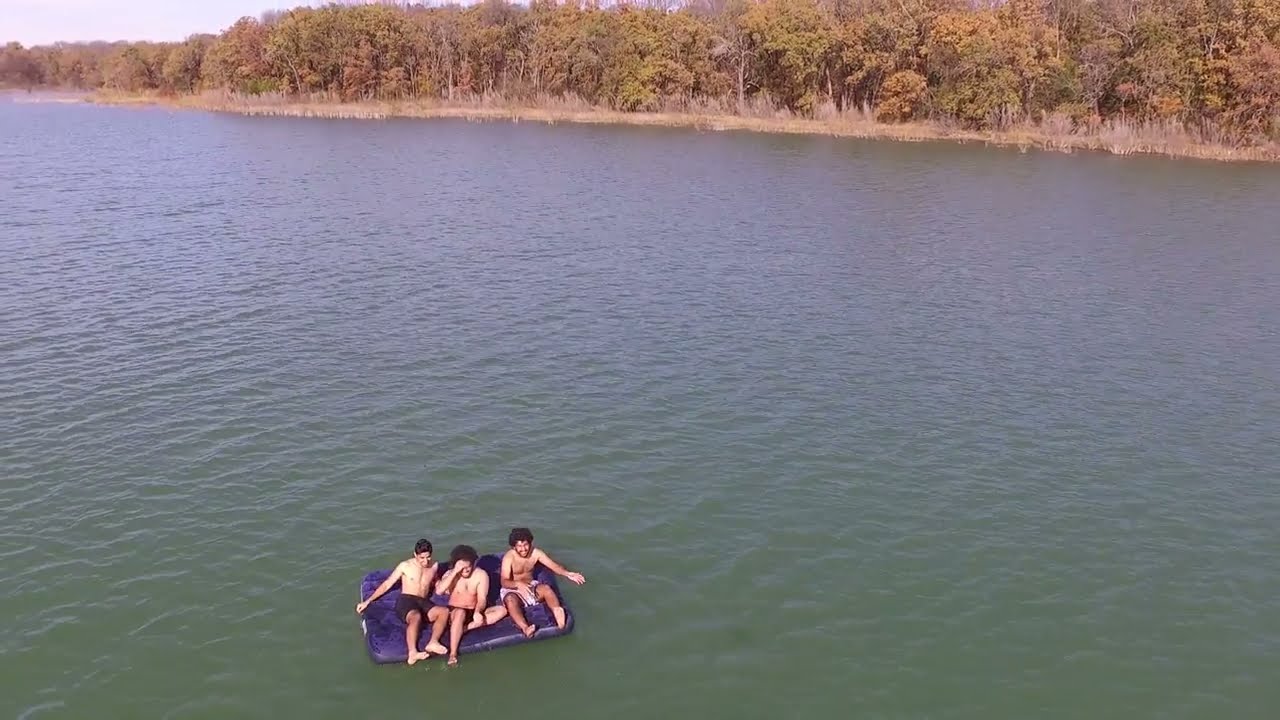The photograph captures three young men or teenagers, shirtless and dressed in swimming trunks, sitting on a purple inflatable raft floating on a bluish, slightly murky lake. The central figure shields his eyes from the bright sunlight, indicating it's a sunny day. The raft is near the center of the image, surrounded by the lake's water, which has a darker tint. In the background, a diverse array of trees showcases autumnal colors—shades of green, yellow, and red—suggesting that fall is approaching. The scene is vibrant with the laughter and smiles of the trio, set against a backdrop featuring the mixed hues of the season and an array of natural elements like bushes, grass, and shrubs lining the shoreline.